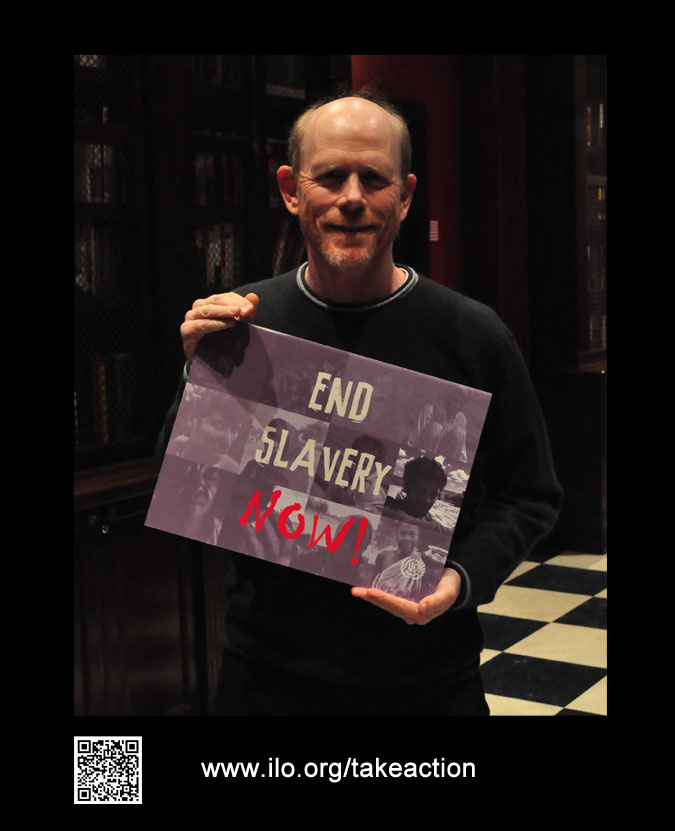This is a close-up photograph of Ron Howard, the director and actor. He is balding, with a thin goatee and a mustache, and is smiling. He is wearing a dark-colored sweater with white trim around the collar and sleeves. In both hands, he is holding up a sign that reads "End Slavery Now" in bold text, with "End Slavery" in yellow and "Now" in red, complete with a red exclamation mark. The sign is also composed of 12 smaller photos creating one larger image of people affected by slavery. At the bottom of the photograph, there is a QR code on the left side and the white text "www.ilo.org/takeaction" on a black background. Behind him, we see a room with a checkered black and white floor, resembling a library with bookshelves that have mesh cage doors.